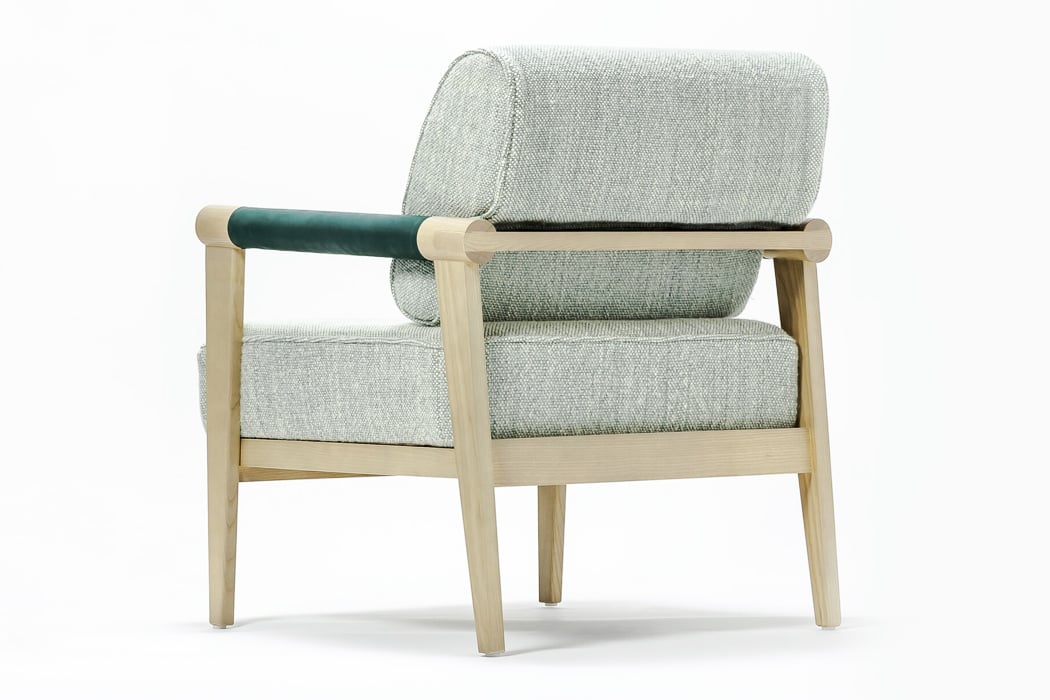The image showcases a simplistic yet classy wooden chair with a light brown finish. The chair features four slender legs and a matching wooden handlebar on the left side, which is accented with a dark green portion. The back of the chair is visible and adorned with a thick gray cushion, complemented by an even thicker cushion on the seat. This elegant piece is set against a plain white background, casting a shadow on the surface below, highlighting its practical and timeless design.